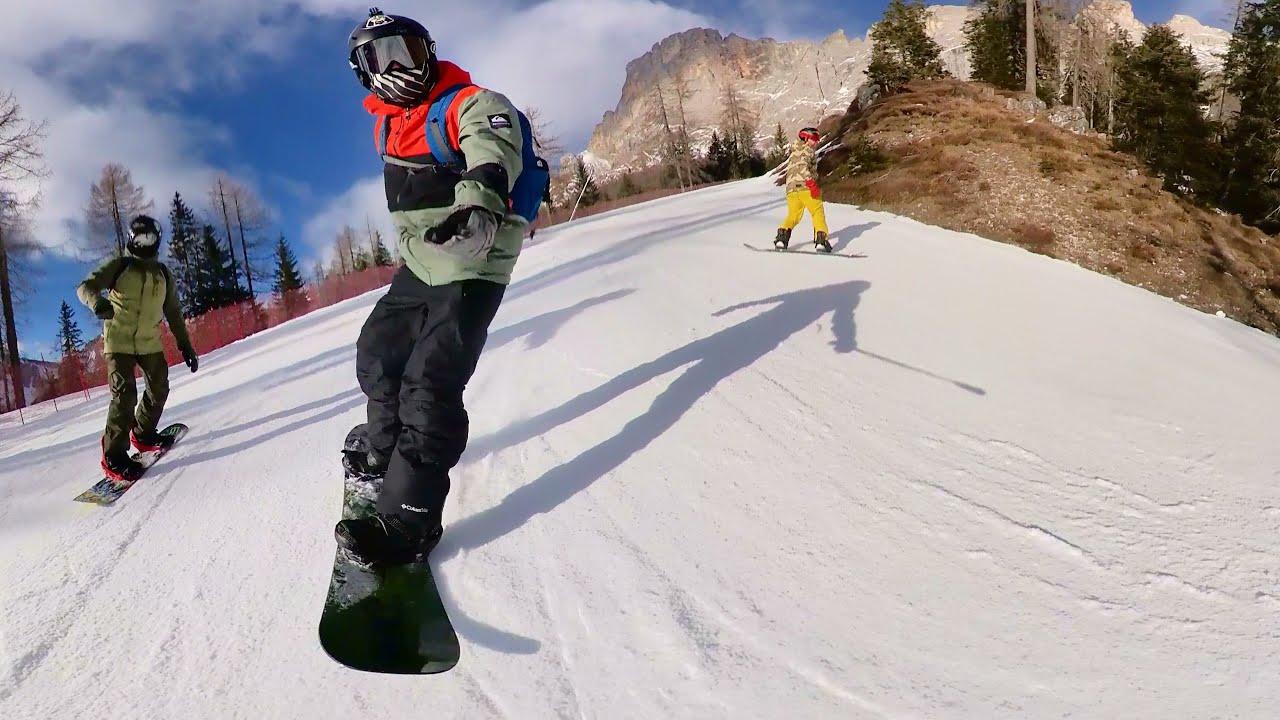The image captures a dynamic scene of three snowboarders descending a snowy, groomed mountain slope directly towards the camera. The photograph is likely taken by one of the snowboarders using a selfie stick, though the stick is cleverly erased, visible only as a shadow on the snow. The central figure, prominently in the middle of the image, is equipped with a gray, black, and red ski jacket, black ski pants, black boots, and a black snowboard. They, like the others, are adorned with a helmet and have a camera mounted on it.

Flanking this main snowboarder to the right (our left) is another rider clad in a brown and black jacket with matching brown pants, and they sport a dark-colored snowboard. To their left (our right), yet another snowboarder is partially turned away from the camera, distinguished by yellow pants and a black and white, or brown and white camo jacket, also wearing a helmet with a mounted camera. Their snowboard runs in the opposite direction toward the edge of the shot.

Backdrop details reveal a clear blue sky with puffy white clouds, scattered patches of exposed rocky ground, and areas densely populated with green trees. A protective snow fence lines portions of the slope, and additional mountain regions and pine trees are visible in the background, indicating a bright and sunny day. All snowboarders are also seen with masks and goggles, further hinting at the brisk and exhilarating nature of their downhill adventure.